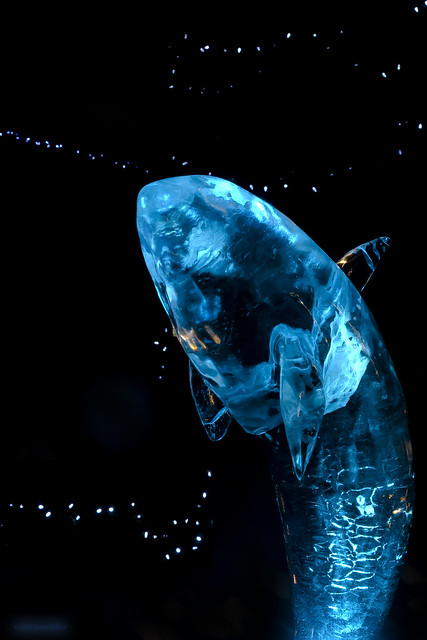The photograph features a predominantly black background dotted with scattered white lines and spots, resembling either lights or bubbles. The centerpiece of the image is a strikingly illuminated, translucent blue figure that appears to be a marine animal, perhaps a shark or a whale, though its exact identity is ambiguous. This figure, positioned in the lower left and extending toward the middle, resembles an ethereal ice or crystal sculpture, glowing with gradients of light and dark blue. Its body curves gracefully, with notable fins on either side— the right fin being lighter in color and the left fin darker and more arched. The entire scene feels reminiscent of an ice sculpture exhibit set against a stark, contrasting backdrop, enhancing the glowing, reflective nature of the creature.